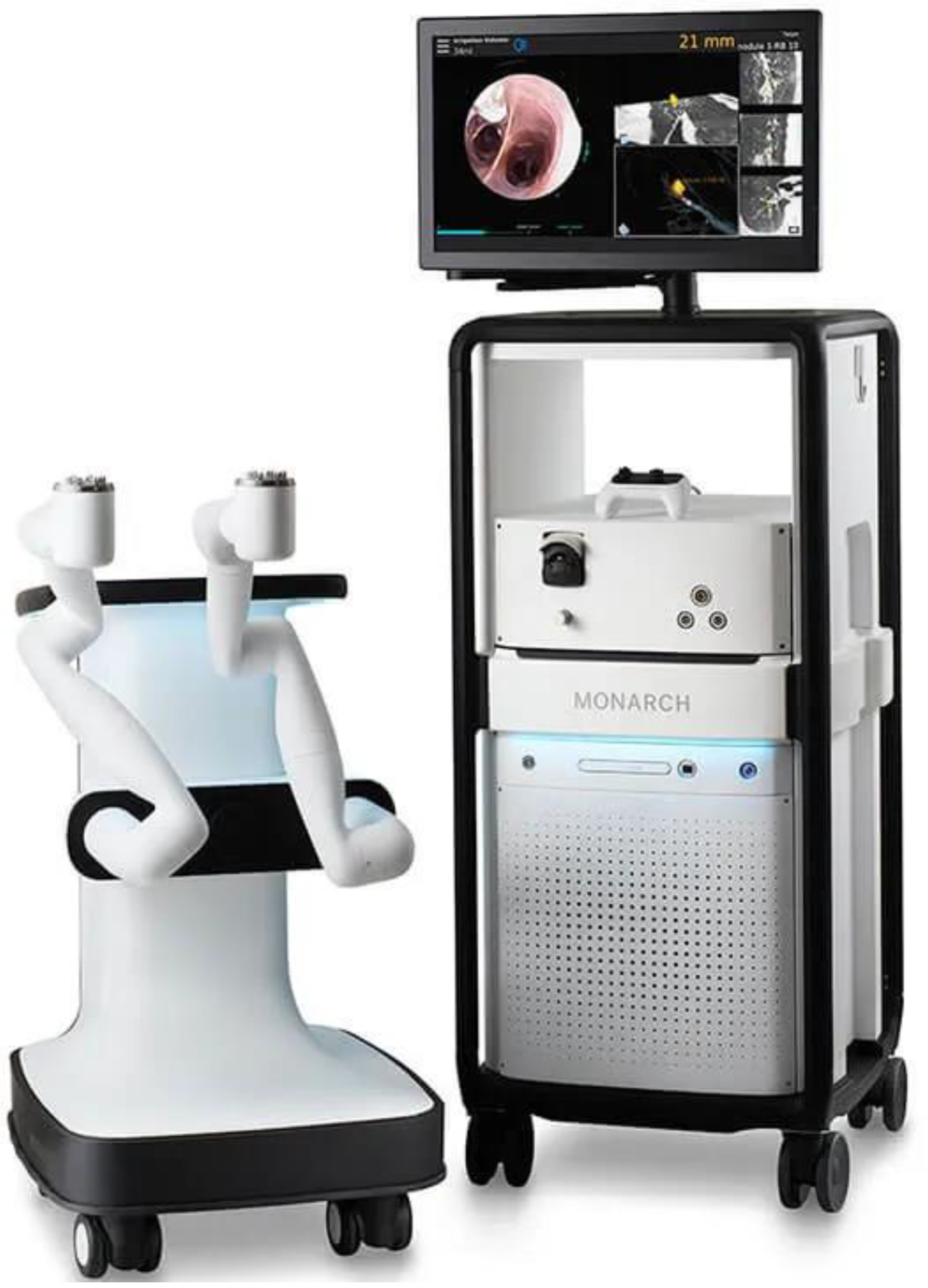The vertically aligned rectangular image showcases a sophisticated arrangement of medical equipment. On the right side, a black, tall rectangular stand with wheels at the bottom supports a small computer monitor at its top. This stand also features a built-in shelf at its base, holding a large white device branded "Monarch," characterized by a vented front and a potential handle or digital display at the top. The monitor, positioned above this Monarch device, displays an image that could be indicative of an internal medical examination, possibly endoscopic in nature.

To the left of this setup, there is another white apparatus, roughly the same height but distinct in design with more curved features. This piece, with a black-accented base and black wheels boasting white centers, has two silver elements protruding from what appear to be cupholders at its top. These protrusions are mechanically complex, resembling gnarled arms or device controls. This left device is robot-like in appearance and stands next to the taller black cart with its integrated medical monitor, creating an intricate and high-tech medical environment.